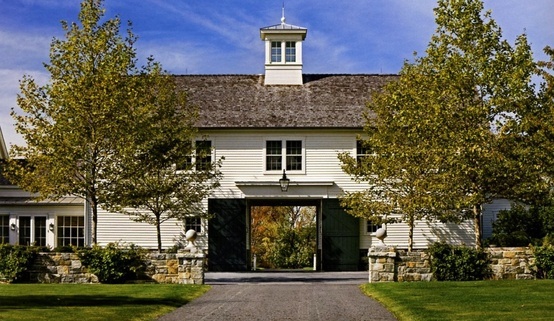This photograph captures a picturesque, sunny day scene featuring a large, converted barn-style garage attached to a house. The garage, which has been entirely repurposed, showcases white siding and a worn, brownish-gray roof with a distinctive white cupola centered on top, standing against a bright blue sky with wispy white clouds. The front of the garage is fully open, revealing an entrance that aligns directly with a back exit, allowing a clear view through to the woods beyond.

The front yard is well-maintained, featuring a freshly mowed lawn on either side of an asphalt driveway that leads up to the garage. A charming stone wall, roughly three to four feet high, borders the grass, with large trees standing majestically on either side of the stone wall, their heights surpassing that of the house. Additional trees and a beautiful green lawn decorate the surroundings, enhancing the serene, natural atmosphere.

Facades of the building exhibit an array of architectural details including multiple windows - five on the front - and an array of secondary doors and windows around the garage. A hanging lamp fixture adorns the front of the garage, adding a quaint touch to the overall scene.